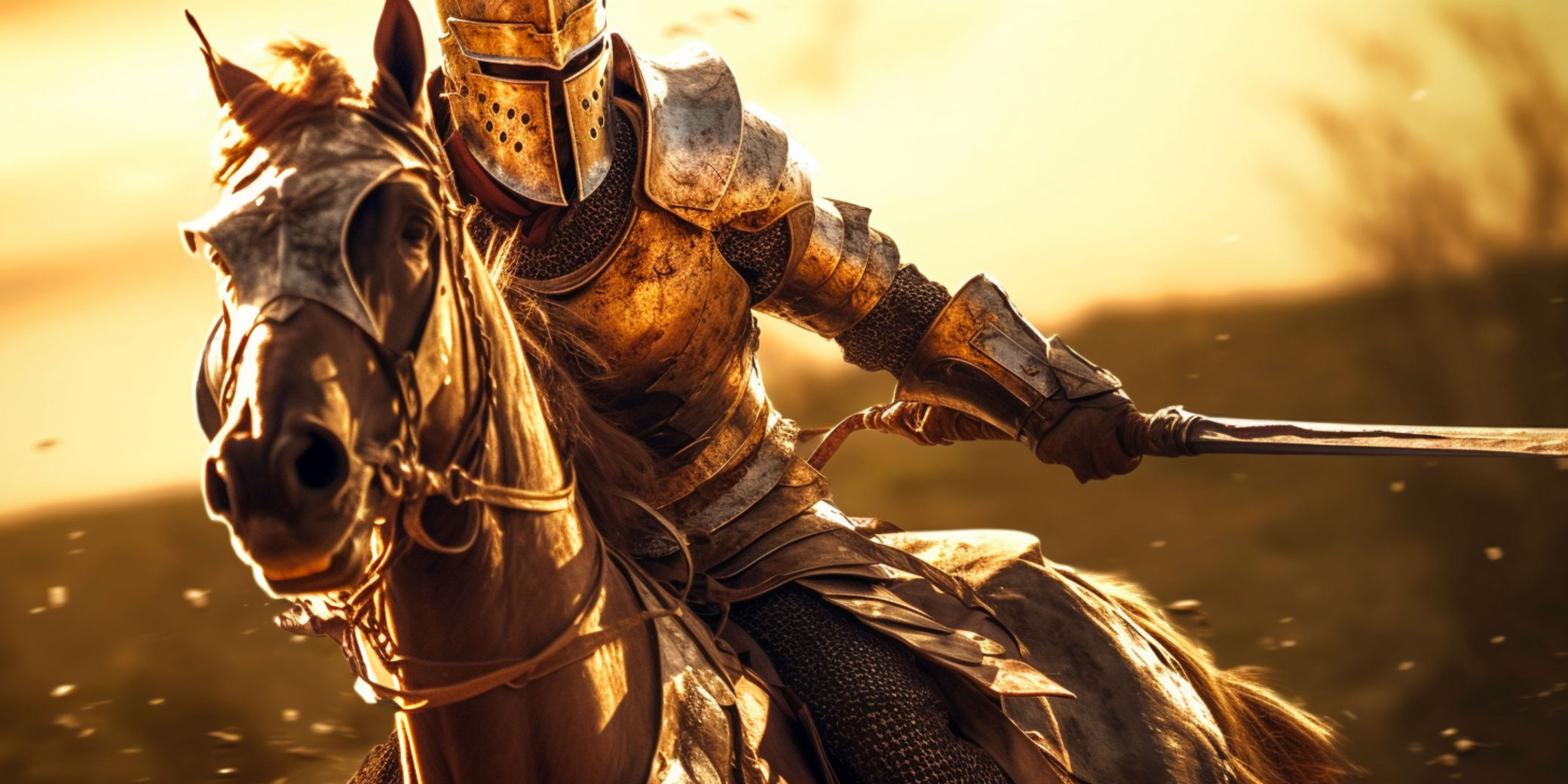In the image, a knight in rust-colored, full-body armor rides a galloping brown horse. The knight's armor features a T-shaped cutout on his helmet for his eyes and mouth, with small, black ventilation holes on the cheeks. His chest and shoulders are clad in layered gold armor that extends down to his heavily armored forearms and gloved hands. Leaning to the left, the knight extends his left hand to the right, holding a sword that goes off the picture’s edge. The knight’s horse is adorned with facial armor, including a shield-like cover between its eyes and a bridle running down its cheek. The horse's mouth is slightly open, revealing a hint of pink, and its nostrils are flared as it kicks up dirt in its wake, indicating its galloping speed. The image, possibly an illustration or computer animation, has a blurred background with a yellow haze at the top and brown at the bottom, emphasizing the motion and fast pace of the scene.